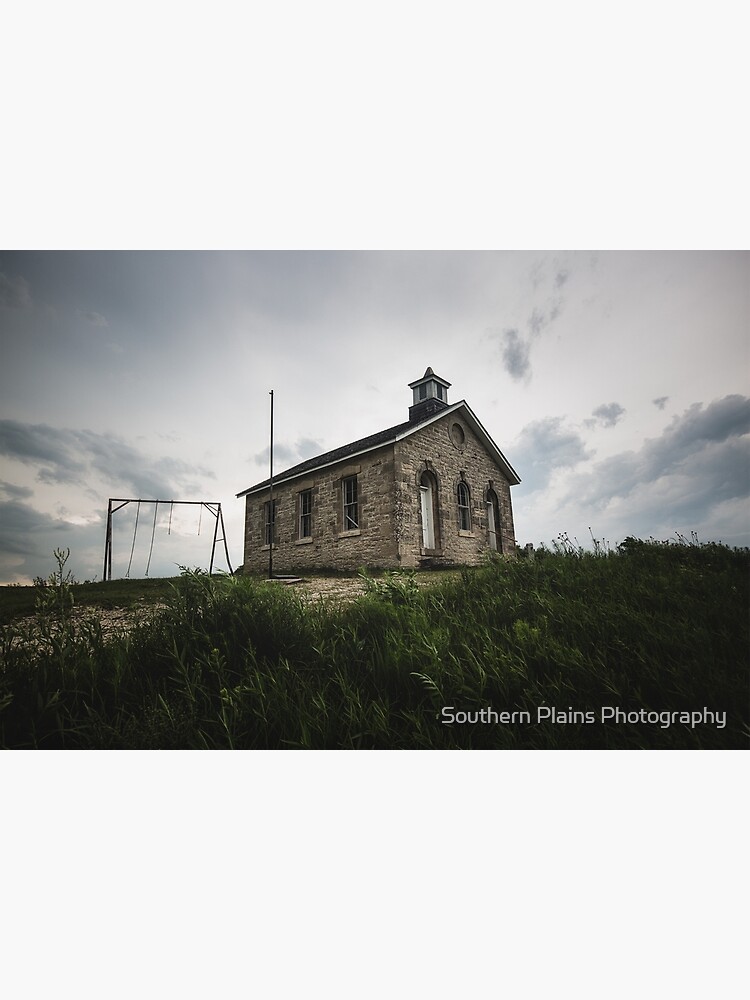This photograph by Southern Plains Photography captures the serene yet desolate scene of a rural brick church, resembling a small schoolhouse or church, resting atop a slight rise. The sky above is filled with dark, swirling clouds in shades of blue-gray, suggesting it's late in the afternoon or early evening. The building features a tiny steeple and a distinct circular window on its front, with three rectangular windows visible along its side. An arched doorway and another arched window adorn the front of the structure. To the left, there's an old flagpole without a flag and a broken swing set standing lonely, adding to the image's melancholic tone. Surrounding the church, a dirt path meanders through short shrubs and tall green grass swaying in the breeze. The watermark of Southern Plains Photography is evident at the bottom right of the picture, anchoring the quiet, wistful moment captured in this rural scene.